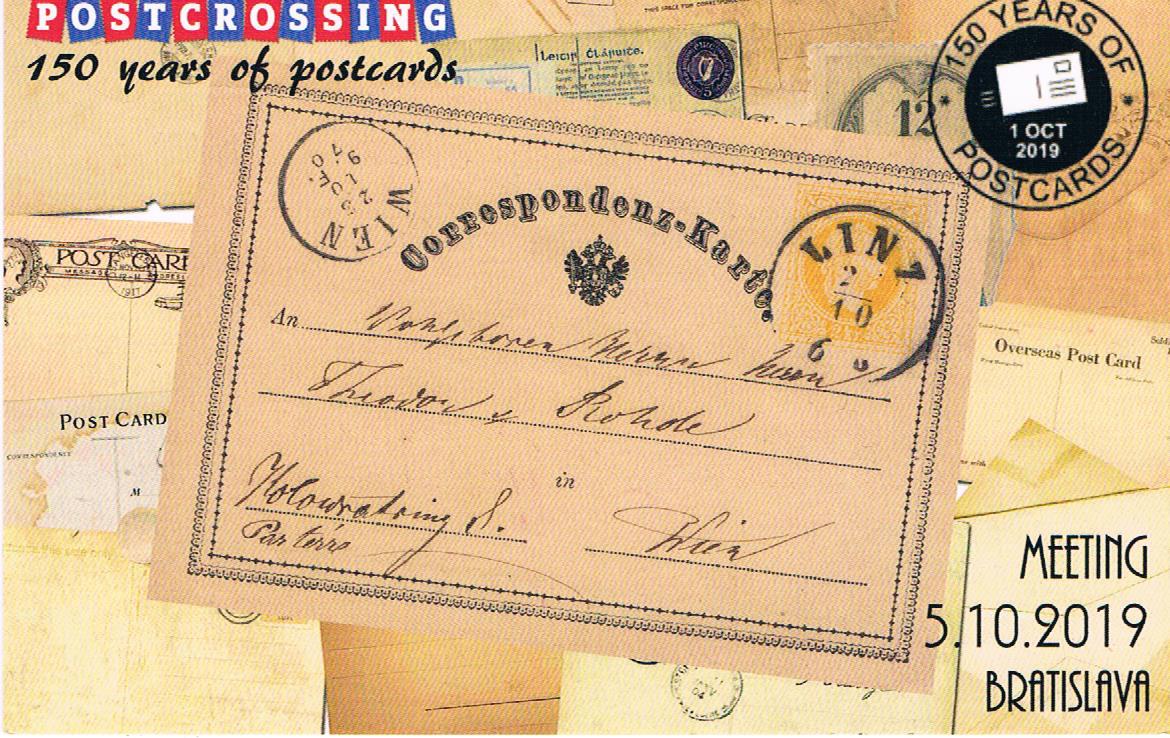The image is a collage centered around a prominent, light brown postcard celebrating "Postcrossing: 150 Years of Postcards." The postcard, framed by a black border, features a mix of elements including a curved black text at the center with the words "Correspondence" and "Cartier" above an emblem resembling an oval shield with wings and a crown. The left and right sides of the postcard are marked with circular postmarks, and a yellow stamp is positioned at the top right. Below the stamp, in strong cursive handwriting, are several lines of text, difficult to decipher. In the bottom left corner appears to be a signature, while the lower right corner contains more cursive writing reading "Meeting 5.10.2019 Bratislava." 

The top left of the image features "Postcrossing" in alternating red and blue squares and "150 years of postcards" below in black cursive. Additionally, the top right displays a black circle with the text "150 years of postcards" encircling a white rectangular silhouette of a letter, dated "1 Oct 2019." Surrounding the central postcard is a background collage of various other brown and cream-colored postcards, suggesting different cities and eras. This jumbled assortment enhances the vintage and commemorative theme of the postcard image.